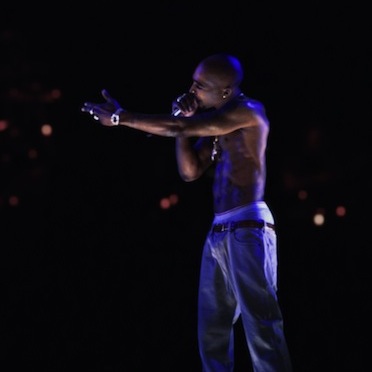The image captures a shirtless, bald black man, who strongly resembles Tupac Shakur, performing on stage, suggesting he is a contemporary singer, possibly a rapper. He has an athletic and well-defined physique, with visible tattoos on his chest and abs. Positioned in a dark, blacked-out background interspersed with scattered white lights, likely from fans’ flashlights or cell phones, the scene exudes the ambiance of a live concert. The singer is adorned with a golden chain necklace, a golden earring, and a silver watch on his left wrist. He is holding a microphone close to his mouth with his right hand while extending his left arm outward towards the audience. He is dressed in loose, baggy jeans that sag below his waist, revealing his white boxers. The subtle dark blue lighting accentuates his appearance and movements on stage.